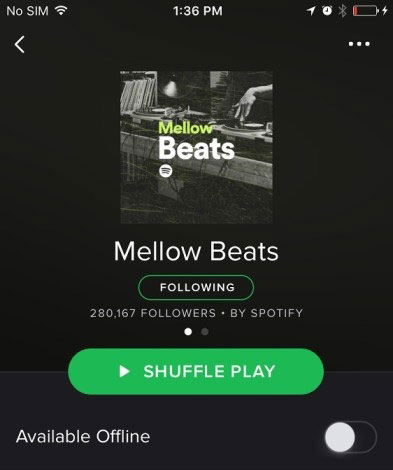This image is a screenshot from the Spotify app, featuring a page dedicated to a music playlist or channel named "Mellow Beats." The background is predominantly black, providing a sleek and minimalist aesthetic typical of Spotify's design. Prominently displayed in the center of the screen, the title "Mellow Beats" appears, indicating the focus of the page. Below the title, there is a label reading "Following," suggesting that the user is currently following this channel. Further down, the text reveals that "Mellow Beats" boasts a substantial following of 280,167 followers, a statistic provided by Spotify.

Beneath this information, a prominent green button labeled "Shuffle Play" invites users to shuffle and play the tracks within the playlist, suggesting an easy way to enjoy the music in a random order. Additionally, at the very bottom of the screen, there is a feature labeled "Available Offline" accompanied by a toggle switch. This switch allows users to enable or disable offline listening, offering flexibility for those who wish to listen without an internet connection. Overall, this detailed view clearly identifies the app as Spotify and highlights the features and user interface elements associated with the "Mellow Beats" channel.